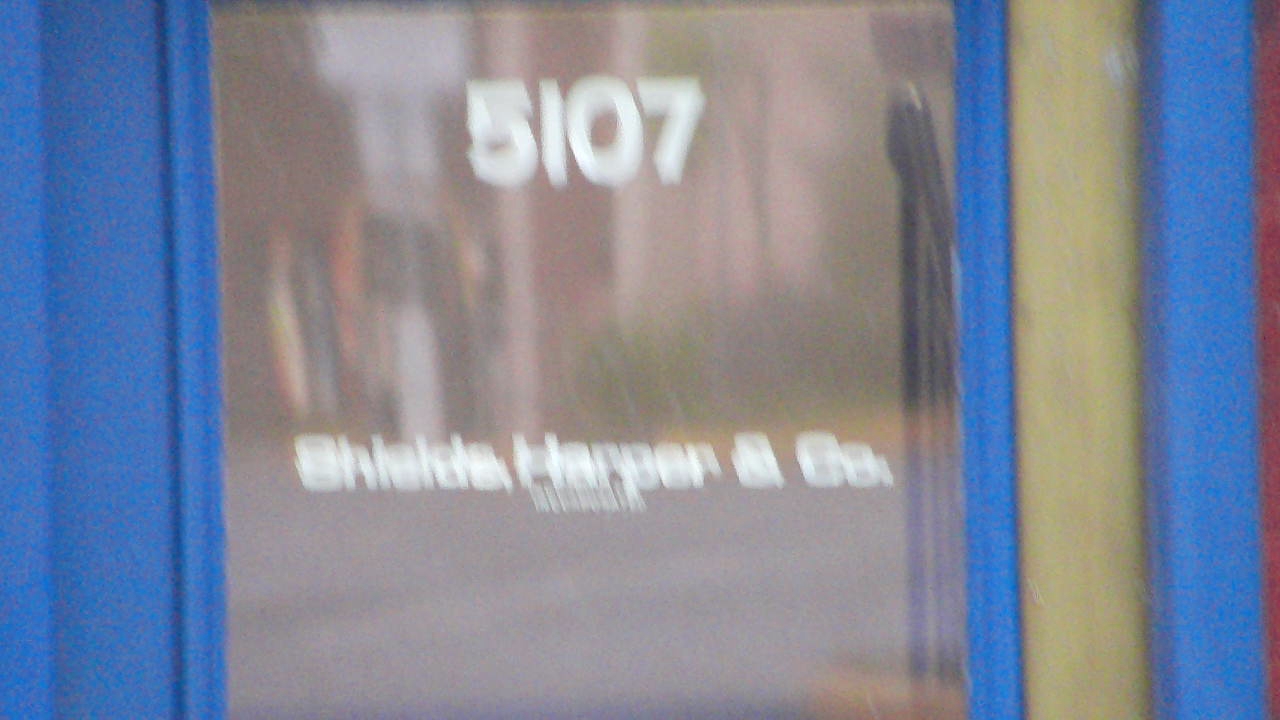The blurred photograph depicts a glass door with a blue frame. The door prominently displays the number "5107" in white lettering at the top, with the words "SHIELDS, HARPER, and COMPANY" below it. Underneath this text, there is additional white text that is too blurry to be discernible. The right side of the image showcases a vertical band of unfinished or beige wood. Reflected in the glass is the scene of an adjacent building, bordered by shrubs and an asphalt surface, possibly a road or parking area. A black handrail's reflection is visible on the right-hand side of the glass. Despite the overall blurriness and out-of-focus nature of the photograph, these details suggest it is the entrance to a business establishment.